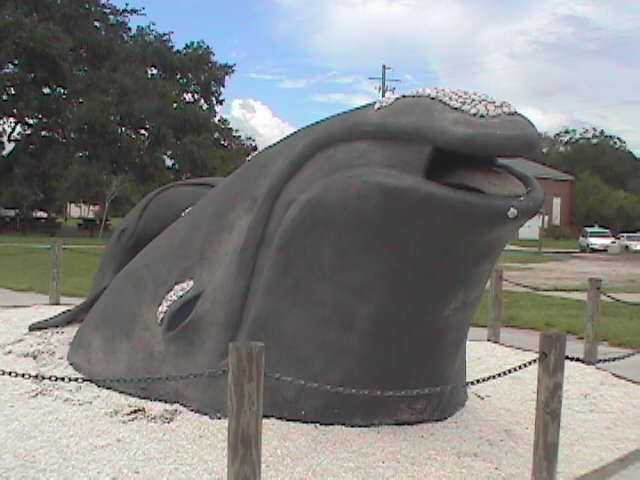The photograph captures a detailed scene centered around a striking statue of a humpback whale’s head breaching from the ground, surrounded by white, grainy rocks resembling sand. Encircling the whale sculpture is a barrier made of short wooden posts connected by chains. The scene is set under a bright daytime sky, which features both blue expanses and various gray and white clouds. In the background, multiple lush green trees stand on the left, while a prominent red brick building with a gray roof is visible on the far right. Adjacent to this building, there appears to be a parking lot with several cars either parked or moving. The overall setting combines natural elements with mild urban surroundings, giving it a picturesque and serene ambiance.